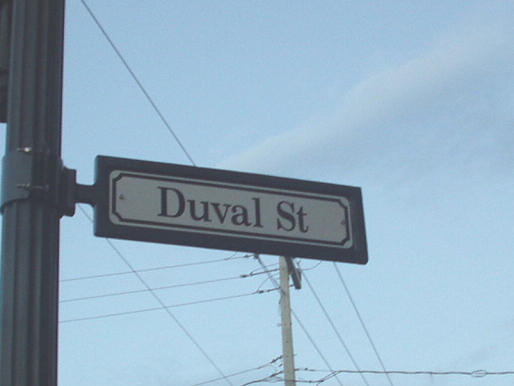This photograph captures a street sign from a low-angle perspective, looking up towards the sky. The sign, attached to a substantial dark gray metal pole, reads "Duval Street" in clear white text on a gray rectangular background. The backdrop showcases a vivid blue sky adorned with fluffy white clouds, creating a picturesque and vibrant atmosphere. Alongside the street sign, a tall wooden telephone pole rises, with telephone and electrical wires extending outwards in both directions, adding an element of urban charm to the scene. The composition effectively blends natural elements with urban infrastructure, capturing a moment of everyday life with great detail and a sense of place.